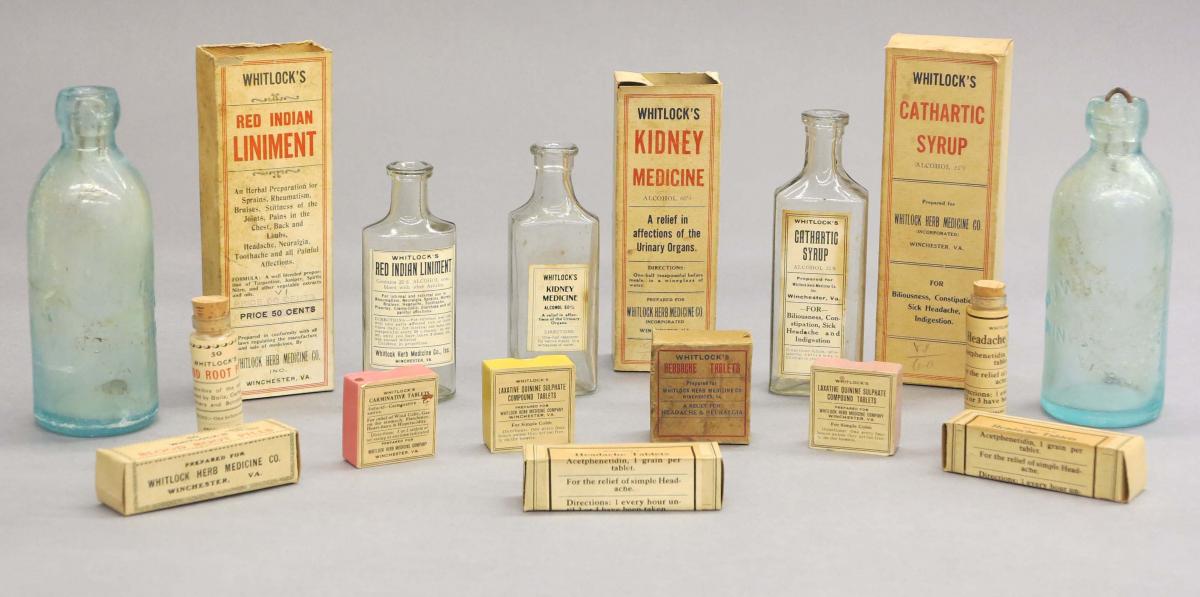The image showcases an antique collection of old-time medicines, featuring an assortment of glass bottles and aged packaging, indicative of their historical period. To the left-most side is a clear blue bottle, mirrored by another clear blue bottle on the right-hand side. Centrally, there are three clear bottles without any blue tint. Adjacent to the left-most bottle is a box labeled Whitlock's Red Indian Liniment, accompanied by a corresponding small bottle. Additionally, the collection includes a Whitlock's Kidney Medicine box towards the middle and a Whitlock's Cathartic Syrup box on the right. The bottles and boxes exhibit significant wear and yellowing, enhancing their antique charm. The larger boxes, marked with titles in red, are placed behind the glass bottles, displaying text like 'Red Indian Liniment' and 'Kidney Medicine,' along with the brand name Whitlock's in black. In front of these larger boxes are several smaller, similarly aged boxes, some obscured, adding to the historical tableau of old medicinal remedies.